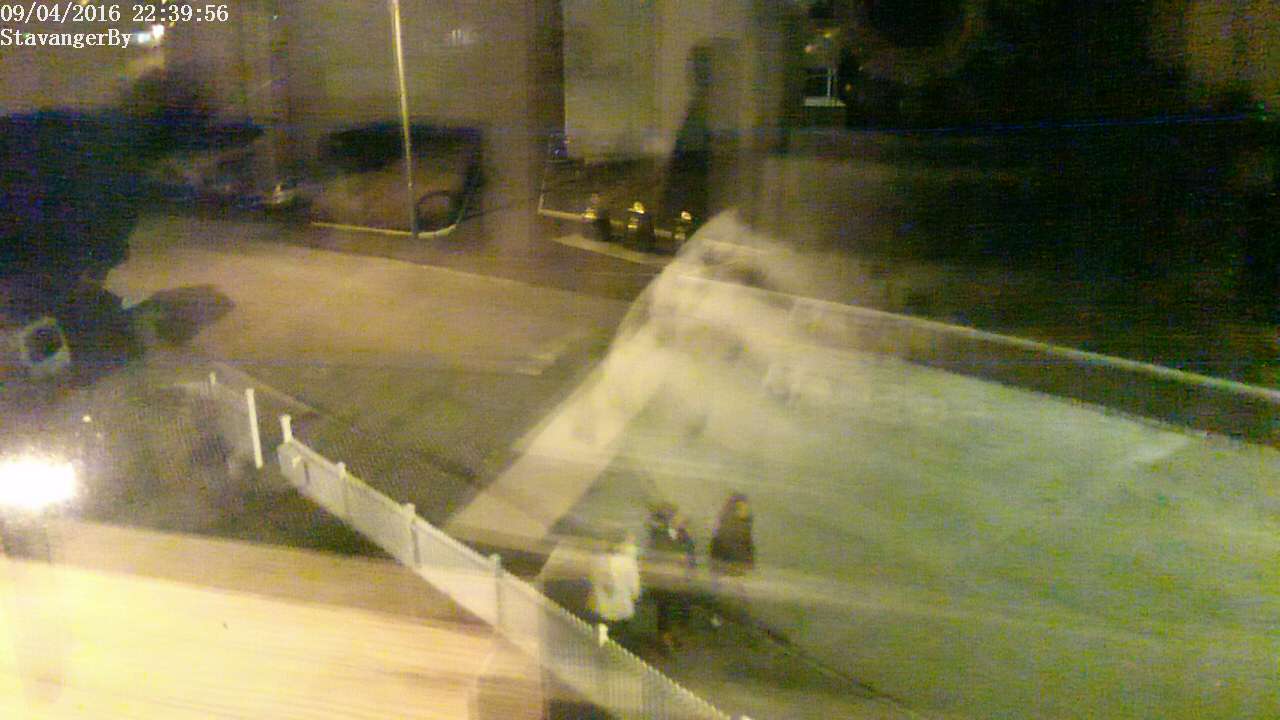The image shows a very blurry and low-resolution scene, seemingly captured through a window with substantial reflections on the glass pane, which obscure parts of the street being photographed. The street, running horizontally with a slight diagonal from the lower right to the upper left, resembles either a bridge with white fence railings or a fenced yard. There are three people visible on the street in the lower half of the photograph, walking to the right—one person in a white coat on the left and two individuals in dark clothing to their right. The far side of the road features some buildings, curbs, and a metal post. Additionally, in the upper-left corner, a watermark can be seen with the date "0904-2016." The overall image quality is poor, with multiple reflections noticeably interfering, including what appears to be the reflection of a lifeless security camera, adding to the confusion in the scene.